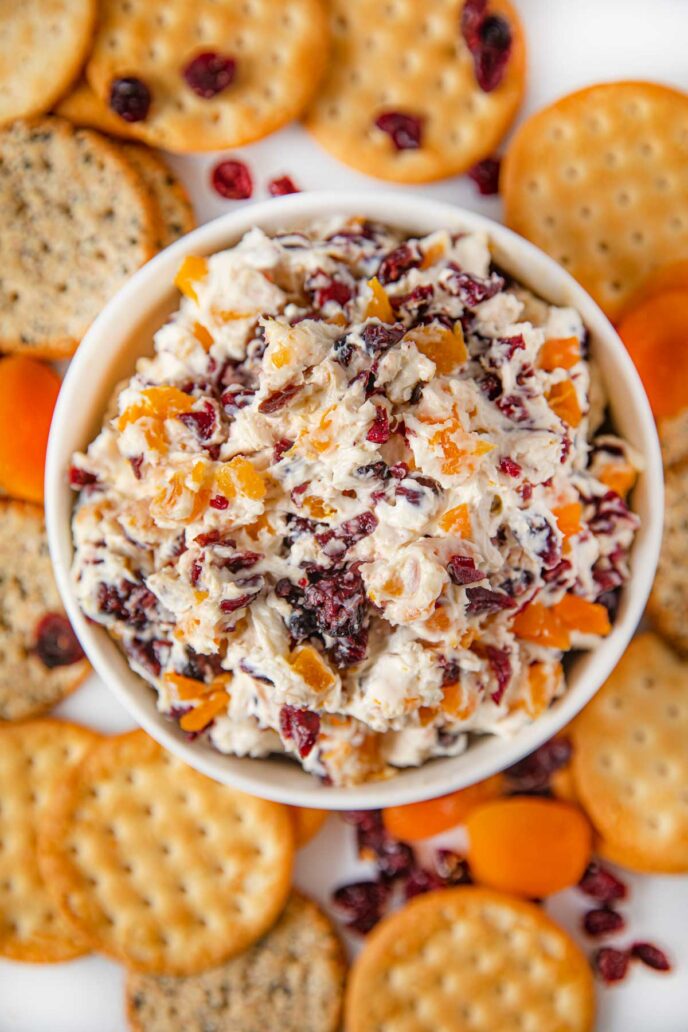This image is a top-down, portrait-oriented view featuring a small white bowl at the center, filled with a creamy, white mixture that resembles vanilla ice cream or a thick dip. The mixture includes visible slices of oranges, likely mandarin oranges, and dark purple or red pieces that appear to be dried cranberries or craisins. The creamy consistency suggests a dairy base, which could be vanilla ice cream or frozen yogurt. Surrounding the bowl are a variety of crackers: Ritz-style round crackers, orange circular crackers with extra holes, and possibly some rye crackers. Additionally, scattered around the bowl and mixed into the creamy mixture are more orange slices and what seem to be apricots. The background appears blurry, but it’s filled with these various crackers and possibly some sliced carrots, adding to the rich mix of textures and colors in the scene.